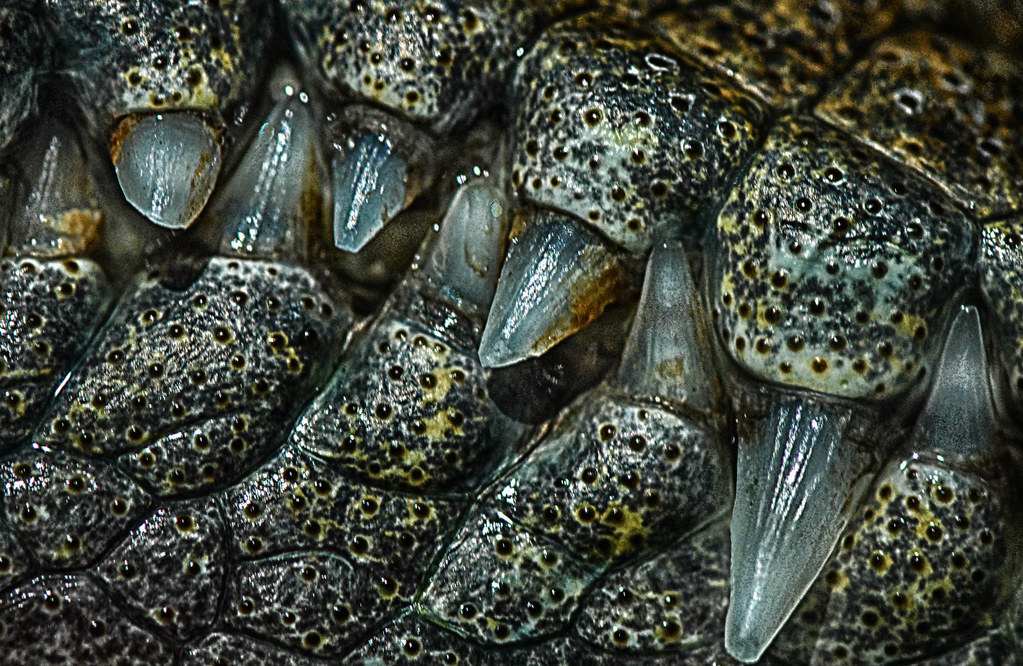This eerie portrait-mode photograph features an extreme close-up of what appears to be reptilian teeth. The interlocking top and bottom sets of teeth, glistening with a white, glassy, and shiny appearance, are tinged with shades of deep blue, grey, dark orange, and gold. The textured gum lines, covered in white-green-yellow scales dotted with black and yellowish spots, enhance the reptilian aesthetic. The teeth, possibly resembling nails due to their intricate overlaps and ridged surfaces, glimmer with a moist, almost icy or glassy quality, lending a surreal and frightening effect to the image.